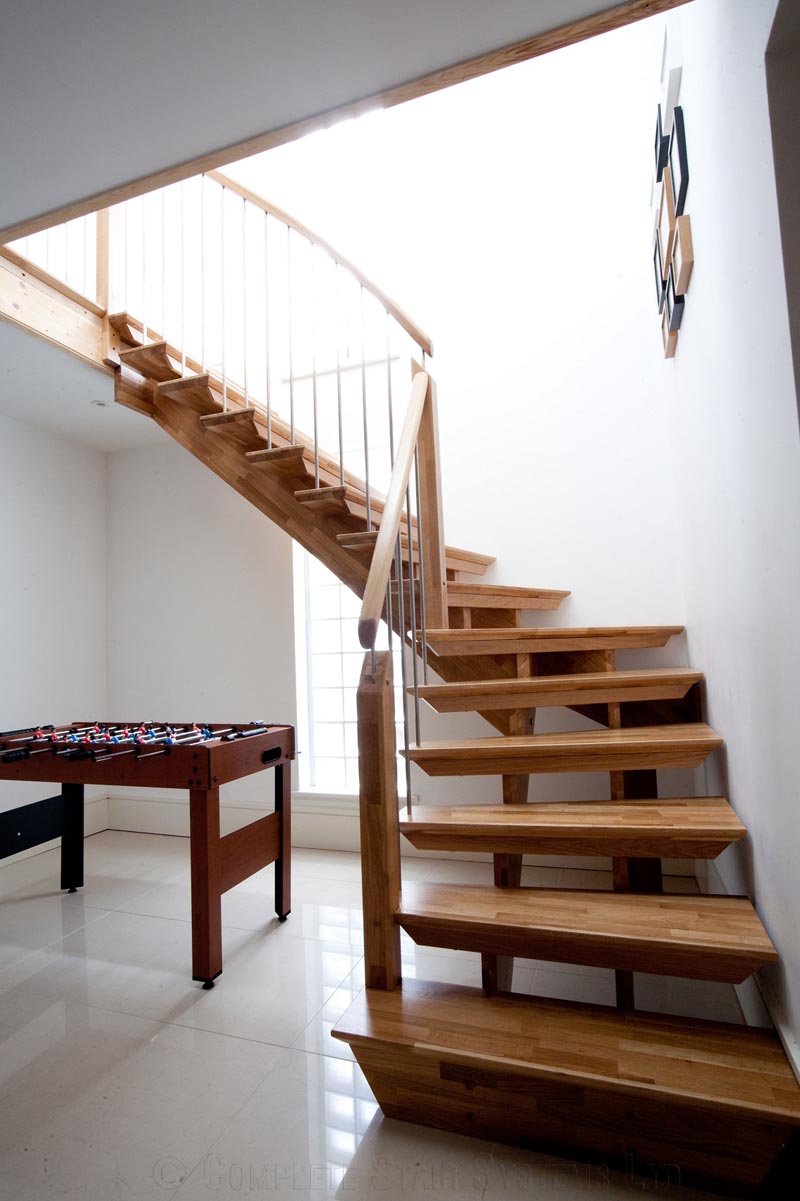The photograph captures the interior of a bright, two-story residential space with a prominent staircase leading to the second floor. The first floor features shiny, reflective white square tiles. The walls and ceiling are uniformly white, creating a cohesive and clean look. Central to the image, the staircase consists of light white wood steps with metal rods for the railing while the tops are adorned with brown wooden sticks. On the right side of the staircase, several picture frames with glass covers are visible, though the images inside are indiscernible; the frames themselves are a mix of black, white, and natural brown wood.

Beneath the staircase is a cubby space housing a brown wooden foosball table with black interiors, equipped with silver rods featuring black handles. The foosball figures are painted red and blue, standing on a white surface. Adding to the brightness of the room, a multi-pane, white-framed window on the far wall under the stairs allows light to flood in, though the view outside is obscured. The overall atmosphere is one of brightness and minimalistic elegance, highlighted by the sleek white surfaces and coordinated wooden accents.